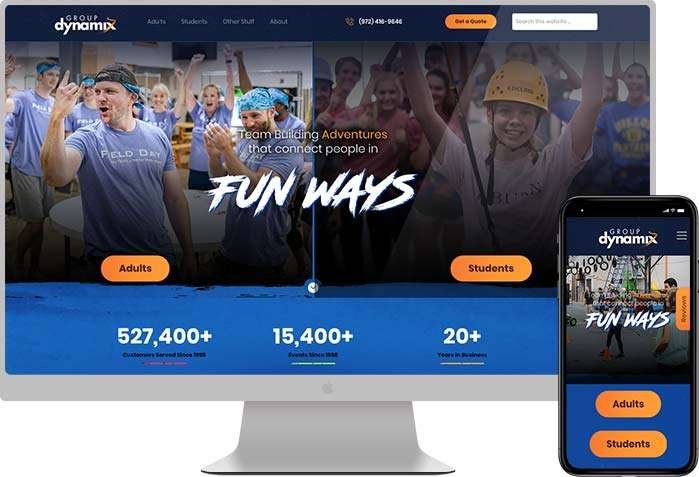The image features a computer and a cell phone placed side by side, both displaying content related to a company named Group Dynamix, spelled D-Y-N-A-M-I-X, with a distinctive design element resembling a snake through the 'X'. The screens highlight various aspects of the company's offerings.

On the left side of the computer screen, there is an image of a group of adults celebrating, all wearing "Field Day" t-shirts and hats. Below this image, there is an orange button labeled "Adults". On the right side, a different picture features students, including a girl wearing a helmet with her arms triumphantly raised. This section is accompanied by an orange button labeled "Students".

The center of the screen prominently displays the slogan "Team building adventures that connect people." At the bottom, there are numerical indicators or sections, leading to more detailed information.

The cell phone screen shows a similar layout but with a different image. It too includes sections for "Adults" and "Students" in orange, maintaining a cohesive and accessible navigation style between both devices.